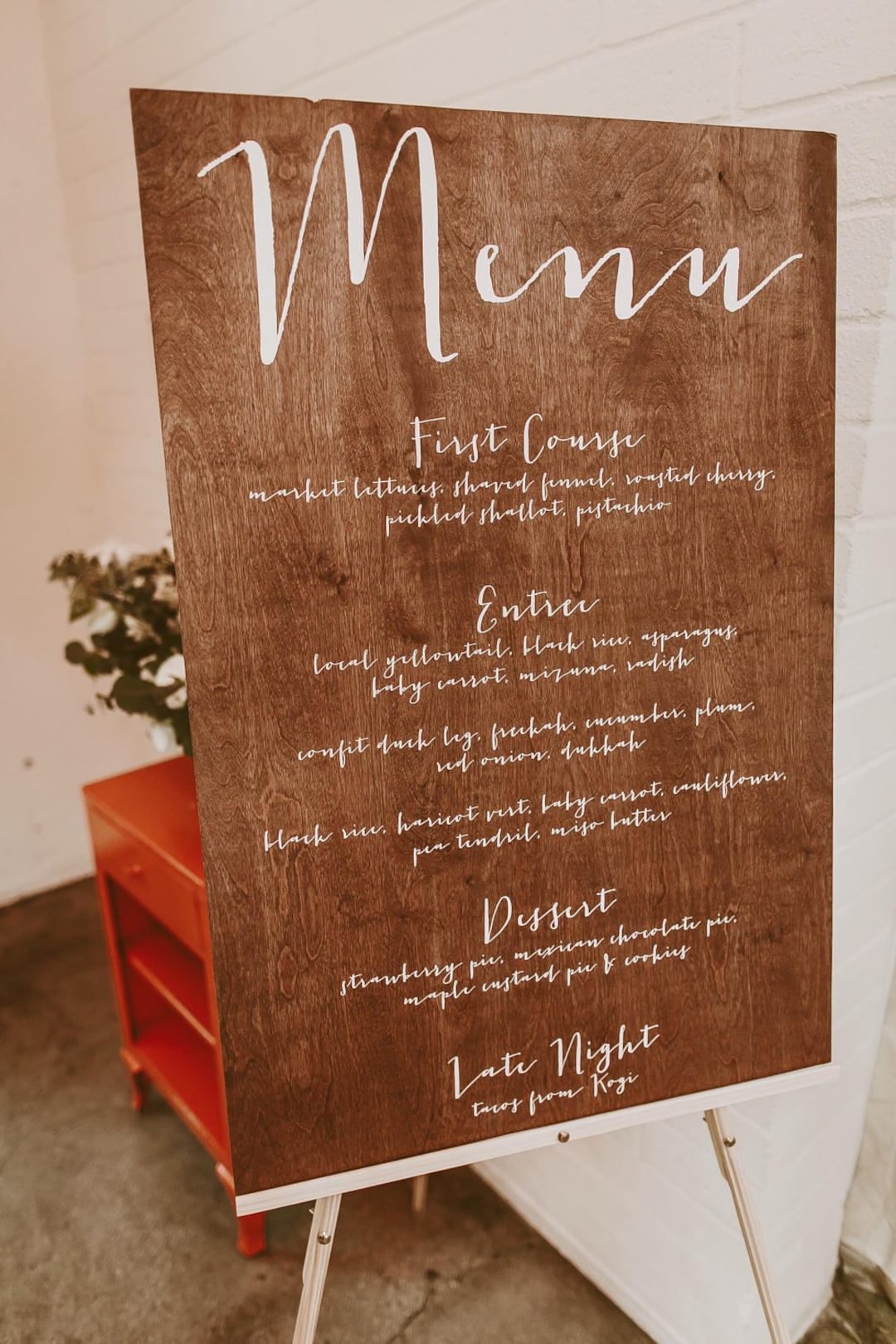This is a color photograph taken indoors of a large, vertically-oriented brown wooden sign on a tripod stand. The sign, featuring a stained wood finish with visible wood grain, prominently displays the word "MENU" at the top in large, white, highly stylized letters. The detailed panel outlines various courses in cursive writing. It starts with "First Course" listing options such as "market fritters, shaved fennel, roasted cherry," followed by "Entree" with choices like "yellowtail, baby carrot." The dessert section includes "strawberry pie, chocolate pie, maple custard pie, and cookies." Below these sections, the word "Late Night" appears. The background features a white wall and a red end table with a plant on it. The floor appears to be brown, possibly made of marble.